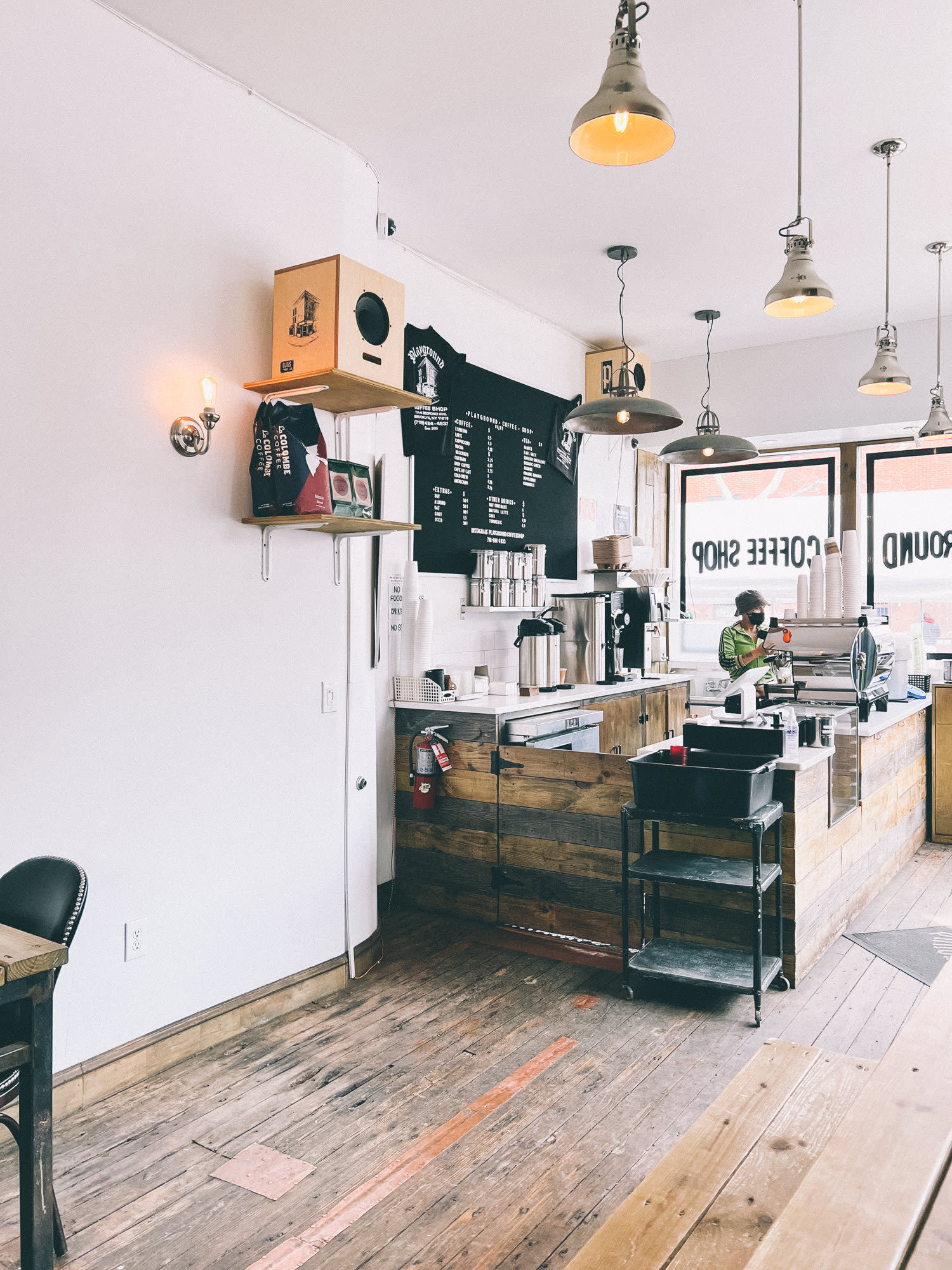This color photograph, taken during the daytime, artistically captures the interior of a classic coffee shop. The perspective is from inside the cafe, looking towards the large windows with the phrase "coffee shop" written backward, which would appear correctly from the outside. The shop's character is highlighted by its wooden flooring, slightly worn for a touch of charm, and wooden countertops and walls around the ordering counter.

In the foreground, a small part of a table and a stylish leather chair are visible. The ceiling is adorned with six metallic lights, each featuring a yellow bulb. To the left, there is a shelf with a few bags filled with coffee and other items, as well as a radio. A fire extinguisher hangs on the wall for safety.

The centerpiece is the barista, dressed in a green shirt, black hat, and a face mask, busy behind the counter. The barista is framed by a black menu board with white text listing the various drinks, though the specific offerings are indistinguishable. The counter is cluttered with various beverages, coffee cups stacked into small towers, and coffee pots, all contributing to the lively atmosphere. The shop appears empty, with no customers present, allowing an unobstructed view of the wooden decor and cozy ambiance of this quaint cafe.